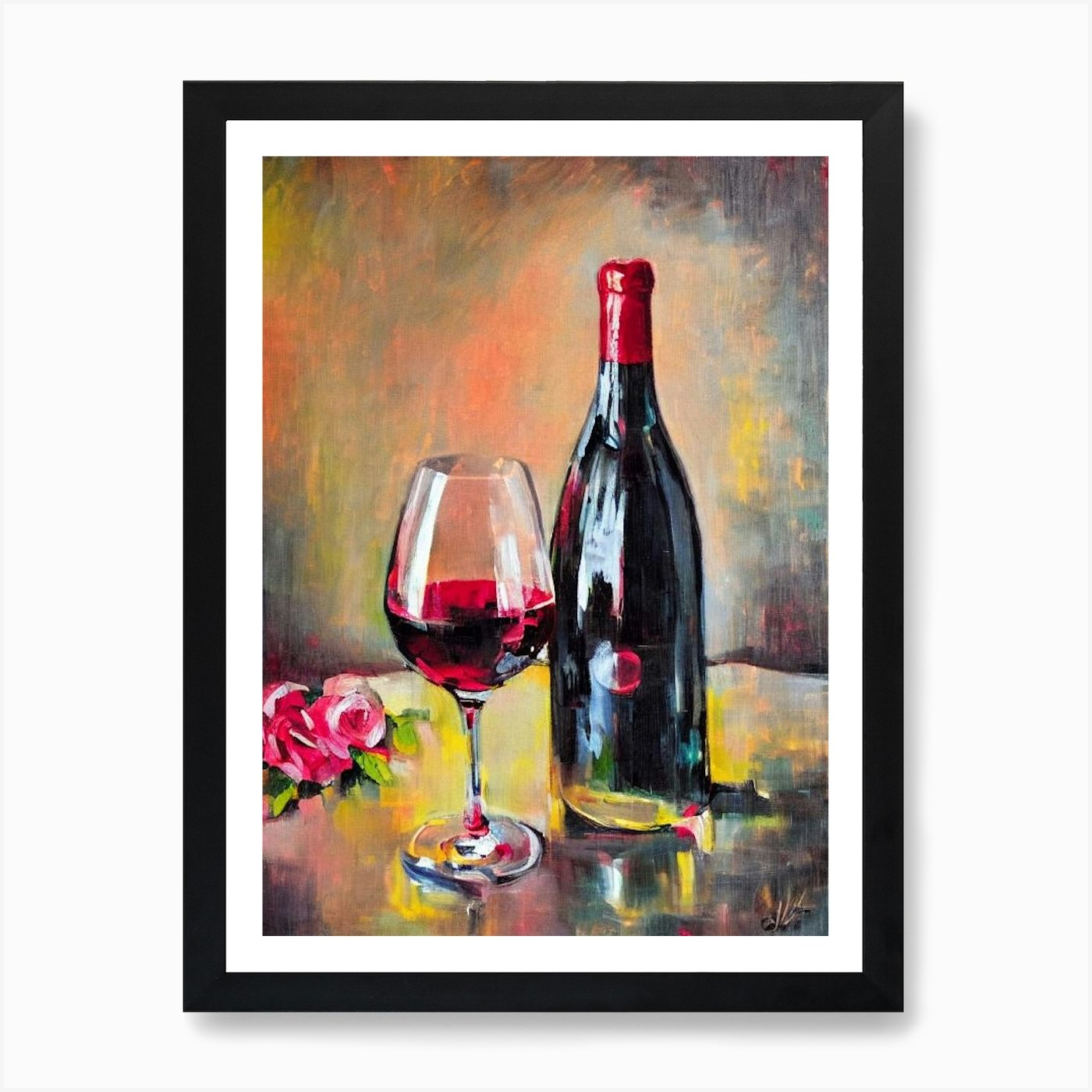This detailed oil painting, set within a black-framed portrait-style design with white matting, captures a still life scene featuring a black wine bottle adorned with a red cork and a red circle on its label. Positioned to the left of the bottle is a clear wine glass, partially filled with red wine, showcasing a thin stem and elegant form. Behind the bottle and glass, a small bouquet of pinkish-reddish roses with leaves adds a touch of natural beauty. The entire arrangement rests atop a clear table, while the multicolored background displays expressive strokes of black, green, yellow, red, orange, and hints of blue, blending harmoniously to complete the composition.